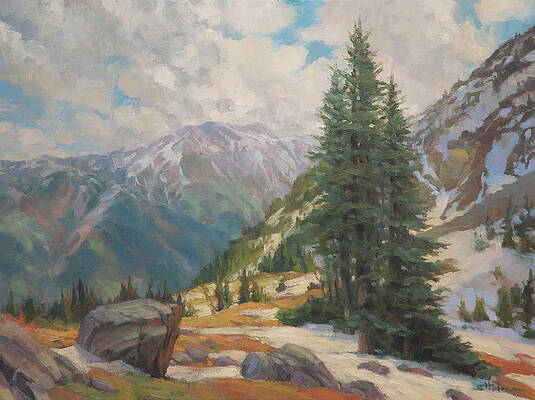This image features a detailed painting of an outdoor mountain scene, capturing the transitional phase when snow has started to melt. In the foreground, several towering and spiky evergreen trees stand prominently, their green-gray hues contrasting against the landscape. Among the trees, there are large, gray boulders with muted peach streaks. Patches of brown dirt and dormant yellowish-brown grass peek through the remaining patches of snow spread across the area. To the right, the lower part of a mountain rises, dotted with rocks and sparse evergreens, and also partially covered with snow. The background showcases distant, snow-covered mountain peaks. The sky overhead is heavily clouded, with sections of white clouds allowing glimpses of blue to peek through, suggesting a cold and cloudy day in this rugged, wilderness setting.